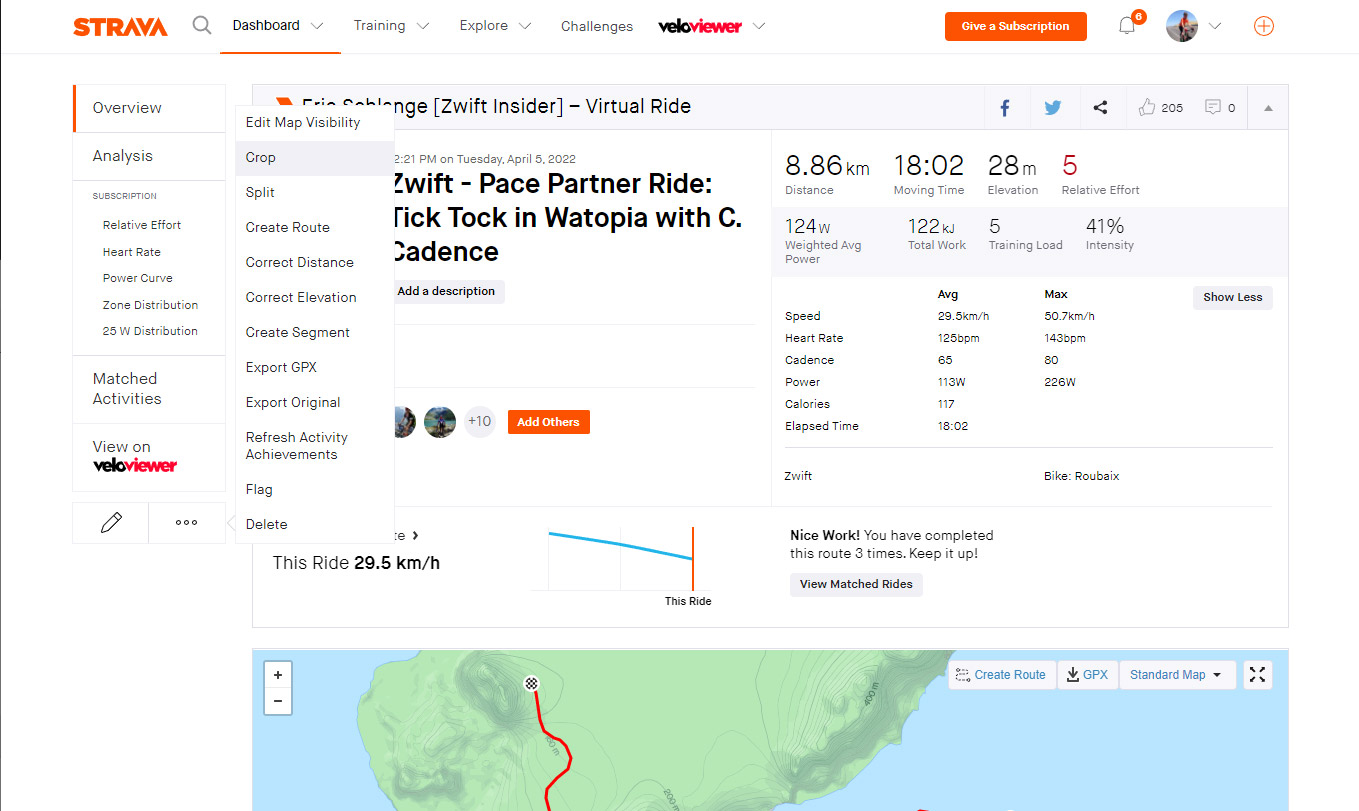This image is a screenshot of a Strava activity page showcasing a virtual ride on Zwift in the Watopia world. You can see the bright orange Strava logo prominently displayed at the top with matching buttons for user interaction. The screen is filled with detailed information about the virtual ride, including metrics such as speed, distance, moving time, elevation gain, and relative effort. Specifically, the rider achieved a speed of 29.5 kilometers per hour, covering a distance of 8.86 kilometers in a moving time of 18 minutes and 2 seconds, with an elevation gain of 28 meters and a relative effort score of 5.

In the top right corner, there's a user icon along with a message area, while the top middle section features navigation tabs like Dashboard (currently active), Training, Explore, and Challenges. On the left side, the Overview tab is selected, with options for deeper Analysis and other dashboard-related features below it.

The bottom part of the page displays a map, indicating the covered route, with additional context provided indicating this is the "C. Cadence" pace partner ride in Watopia. The page also emphasizes the cumulative achievement with a congratulatory note, stating that this route has been completed 21 times by the user. The overall tone of the page is user-friendly and motivational, encouraging continued engagement and progress.